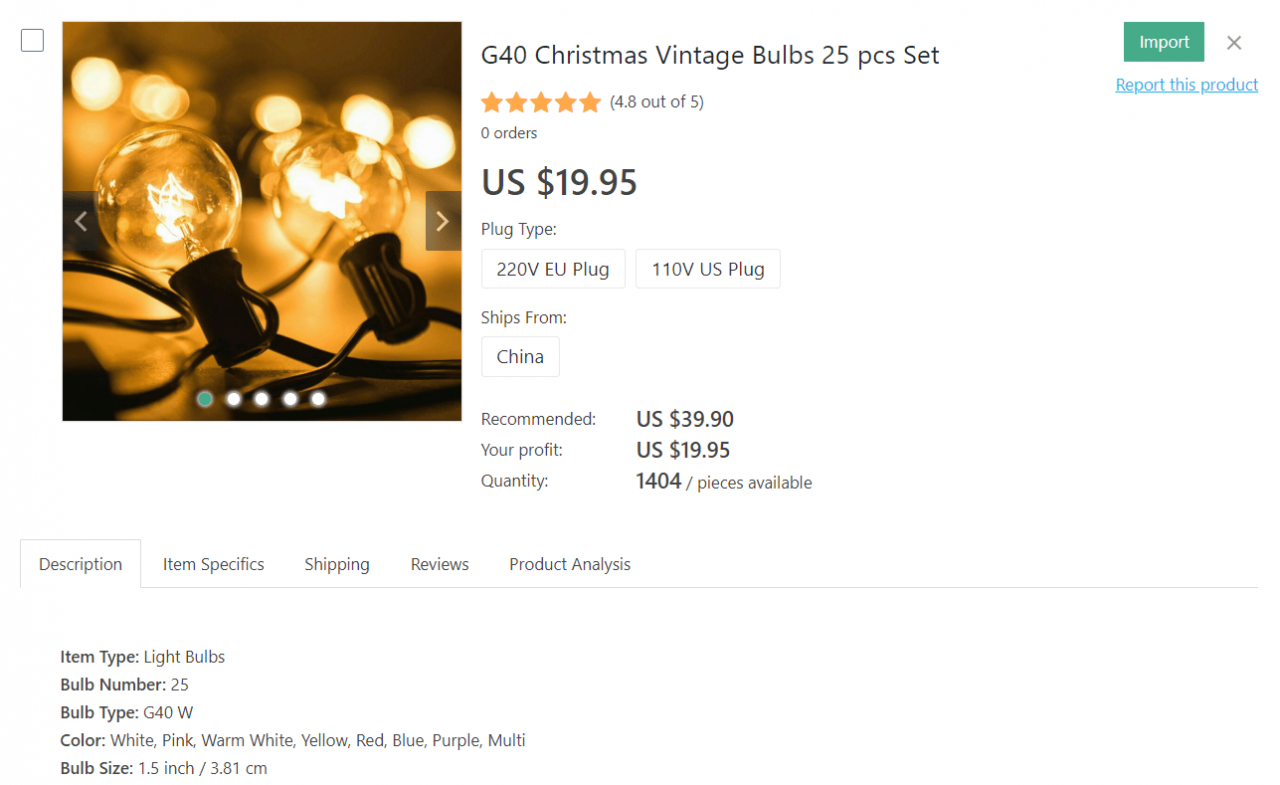This detailed image displays a sales listing for vintage-style G40 Christmas light bulbs. The prominent feature is a pair of almost perfectly spherical, globular light bulbs that resemble classic incandescent lights. These light bulbs are depicted clipped together and connected by two wires, emphasizing their design.

On the right side of the image, a detailed caption provides more information: "G40 Christmas Vintage Bulbs, 25 pieces set," which boasts an impressive rating of 4.8 out of 5 stars, although it currently has zero orders. The price is listed at $19.95 USD. The plug types available for these bulbs are categorized into two options: a 220V EU plug and a 110V US plug, with the items shipping from China.

Below the product details, several tabs offer further information, including "Description," "Item Specifics," "Shipping," "Reviews," and "Product Analysis." Currently, the "Description" tab is shown, featuring attributes such as the item type (light bulbs), the number of bulbs (25), bulb type (G40W), and available colors (white, pink, warm white, yellow, red, blue, purple, and multi). The size of each bulb is specified as 1.5 inches or 3.81 centimeters.

The image also shows that the product is being marketed with a recommendation price of $39.90 USD, promising a profit of $19.95 USD per set. An impressive stock of 1,404 pieces is available for purchase. In the upper right corner, a prominent green button labeled "Import" next to an 'X' is visible for user convenience, along with a blue link allowing users to "Report this product."